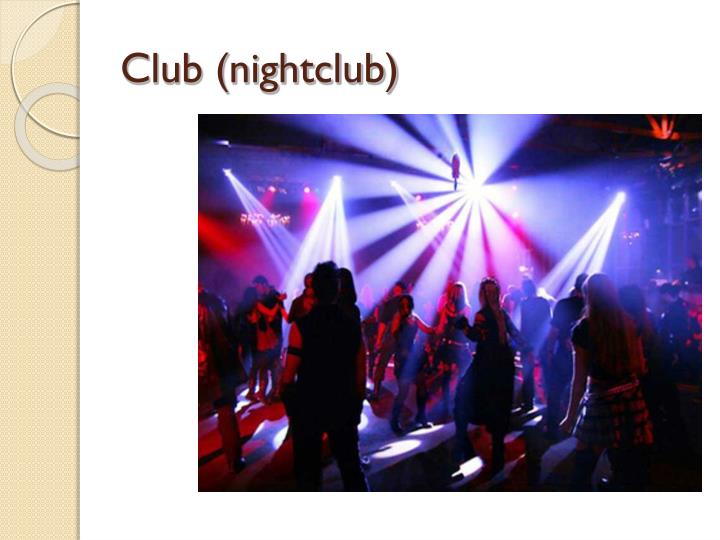The image appears to be from a textbook slide or presentation, featuring a bordered design on the left side composed of a textured or beige strip with two circles at the top—one larger with a thin outline and the other smaller with a thick outline. The main content is placed against a flat white background. At the top of the image, there is a deep reddish-brown text that reads "club," with "nightclub" in parentheses. 

The central photo captures a vibrant nightclub scene characterized by a dark atmosphere illuminated by an array of flashing lights in hues of blue and purple. Light rays reflect dynamically off the dancing crowd, enhancing the energetic ambiance. The crowd consists of people, primarily women, dressed in various stylish outfits. The most prominent individual in the foreground is a young woman with long hair, wearing a black shirt and a black-and-white striped skirt. Overall, the scene showcases a lively night out with people enjoying themselves on the bustling dance floor.